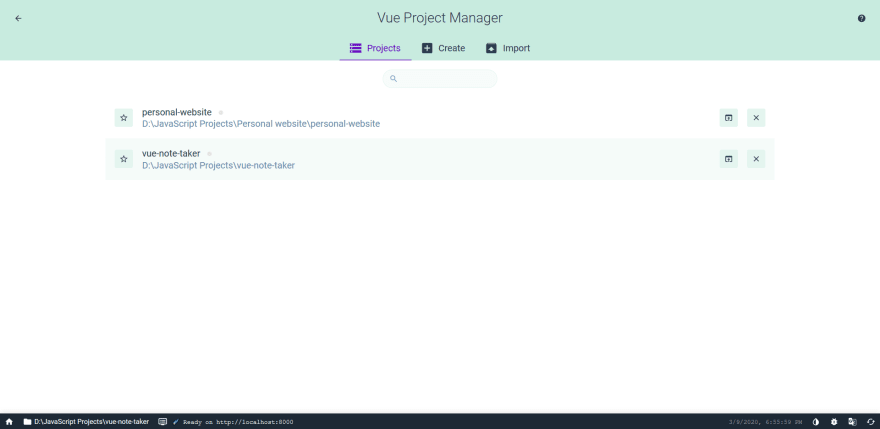In this image, we are looking at a horizontally-oriented screenshot with a pale mint green top banner. Centered within this banner is large gray text that reads, "View Project Manager." Below this top section, there is a menu. On the left side of the menu, there is the word "Projects" in purple text, and to its right, a purple underlined link. Further to the right are two black boxes – one featuring a plus sign labeled "Create," and the other with an upward-pointing arrow labeled "Import."

Below this menu, the background shifts to solid white. In small gray text, there is the label "Personal Website." Underneath this label is a filepath "D:/Javascript Projects/Personal Website/Personal Website," also in gray text. Further down, there is a pale green box with a star icon. Inside this box, in gray text, it reads "View Note Taker." Beneath this text, another filepath is displayed: "D:/Javascript Projects/View Note Taker." 

This detailed and well-structured layout aids in navigating through the different sections and projects in the project management interface.